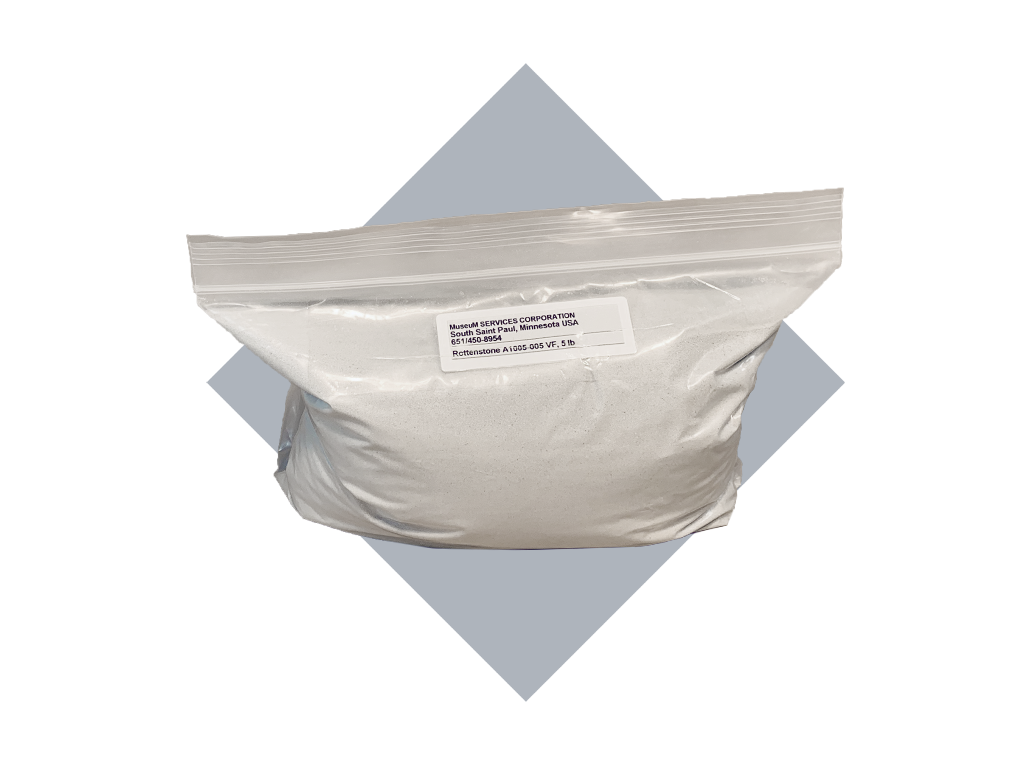This image is a full-color photograph featuring a simple, yet detailed setup. Against a solid white background, there is a medium gray, diamond-shaped figure, reminiscent of construction paper or a baseball diamond base. Positioned diagonally, this diamond provides a backdrop for a heavy-duty, white Ziploc bag that appears professionally sealed and filled with a uniformly distributed white powder. 

The bag prominently displays a bright white label with black text. The label reads "Museum Services Corporation, South St. Paul, Minnesota, USA, 651-450-8954." Additionally, there is a product code "Rottenstone A1005-005VF" and a weight indication of "5 pounds." The image likely has been edited, giving it a scanned appearance with clean edges.